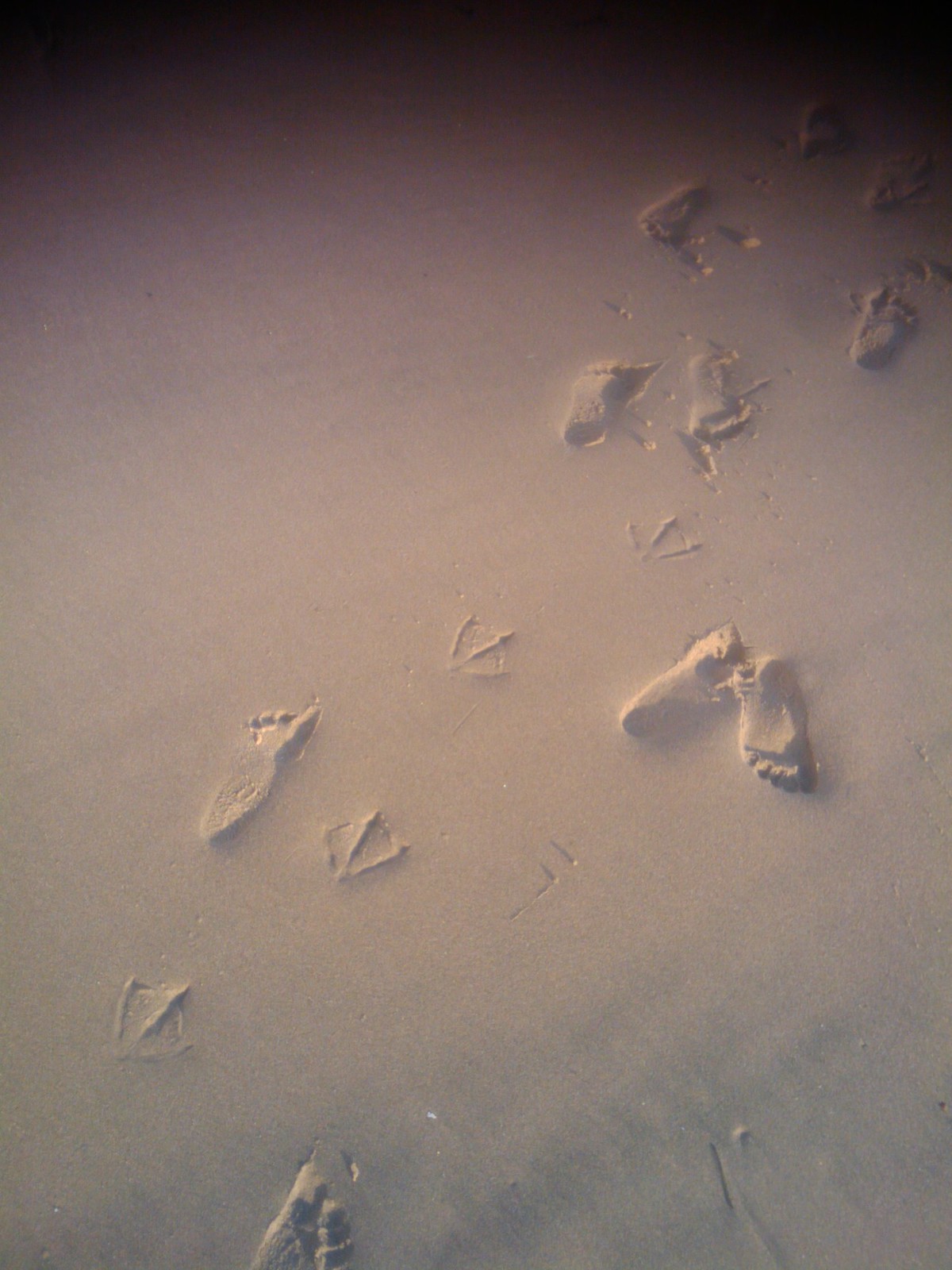The photograph captures a detailed and intriguing scene on a beach with fine, almost pristine, sandy soil that takes on a pinkish hue due to the lighting and white balance of the image. The composition features an intricate pattern of both human and bird footprints, primarily those of a large bird like a goose, crisscrossing each other. Human footprints are clearly visible, moving from the bottom left to the top right of the image and crossing paths with the distinctive bird prints. The sand's beige color subtly transitions into a darker gradient towards the top of the photo, adding depth and contrast to the scene, which is bathed in a soft pinkish, purplish, gray tint, enhancing the dreamlike quality of the moment captured.